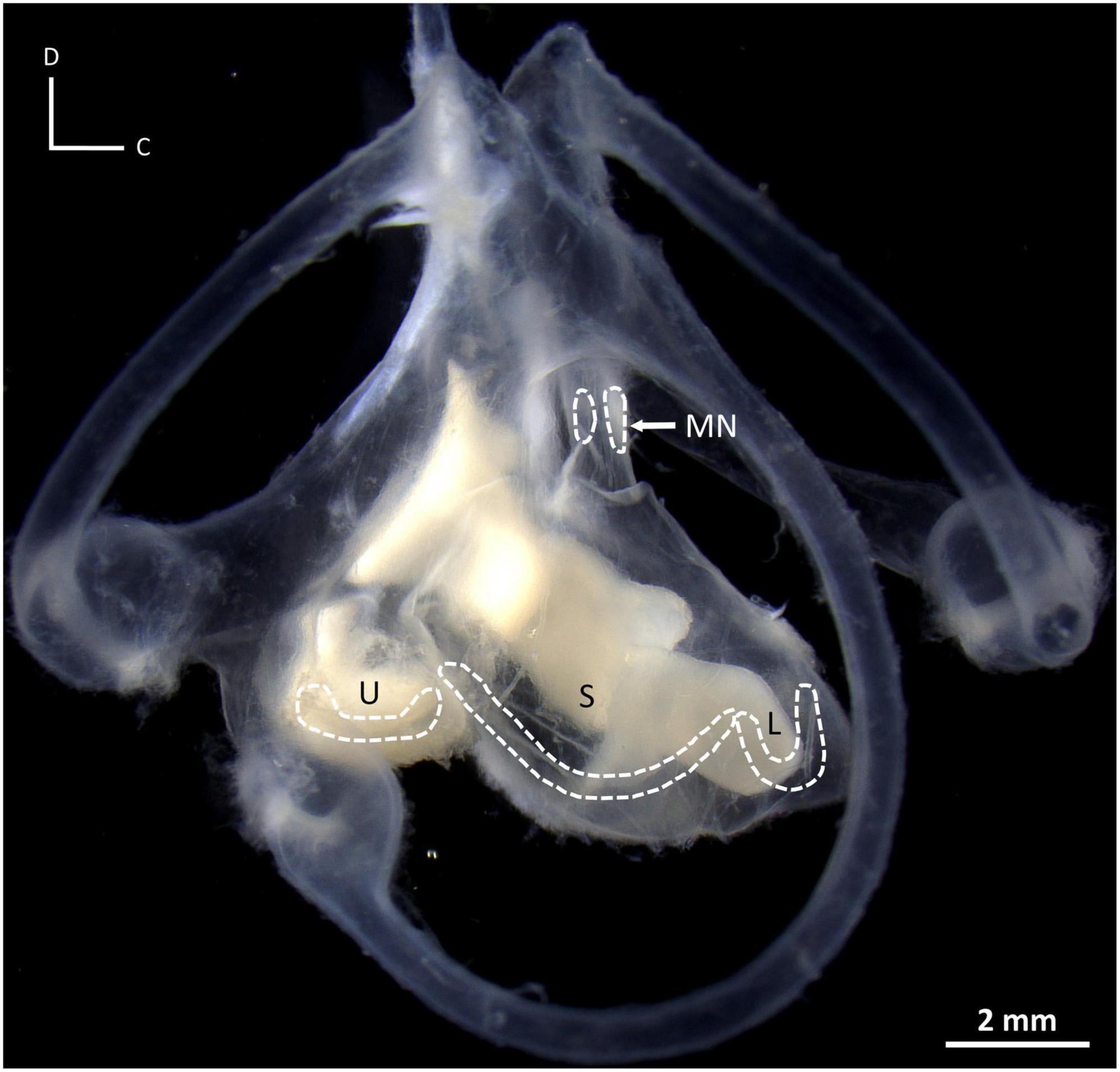This detailed image depicts what appears to be an x-ray or another form of high-resolution imaging, presenting a highly intricate and translucent central structure against a stark black background. The main feature resembles a stem that branches out into four distinct tube-like extensions, each culminating in rounded knobs. Central to the image is a triangular-shaped section containing multiple white blobs, giving it a complex, almost organic appearance.

Marked by an array of fine details, the image features various labeled elements: in the top left corner, the text reads "D and C"; in the bottom right corner, it mentions "2 millimeters," indicating the scale of the object. Additionally, three of the white blobs within the central structure are labeled with letters: "U" on the leftmost blob, "S" in the middle, and "L" on the right, each outlined with dotted white lines, with the "S" resembling a wide 'U' shape and the "L" outlined similarly to a 'J'. Two other white, dotted spots labeled "MN" sit atop the stem leading to this central blob.

The entire structure within the image is composed of a grayish, smoky hue, and visually, it bears a resemblance to wavy tubes or perhaps an abstract interpretation of organic matter or microscopic life forms, reinforcing its enigmatic and minute nature.